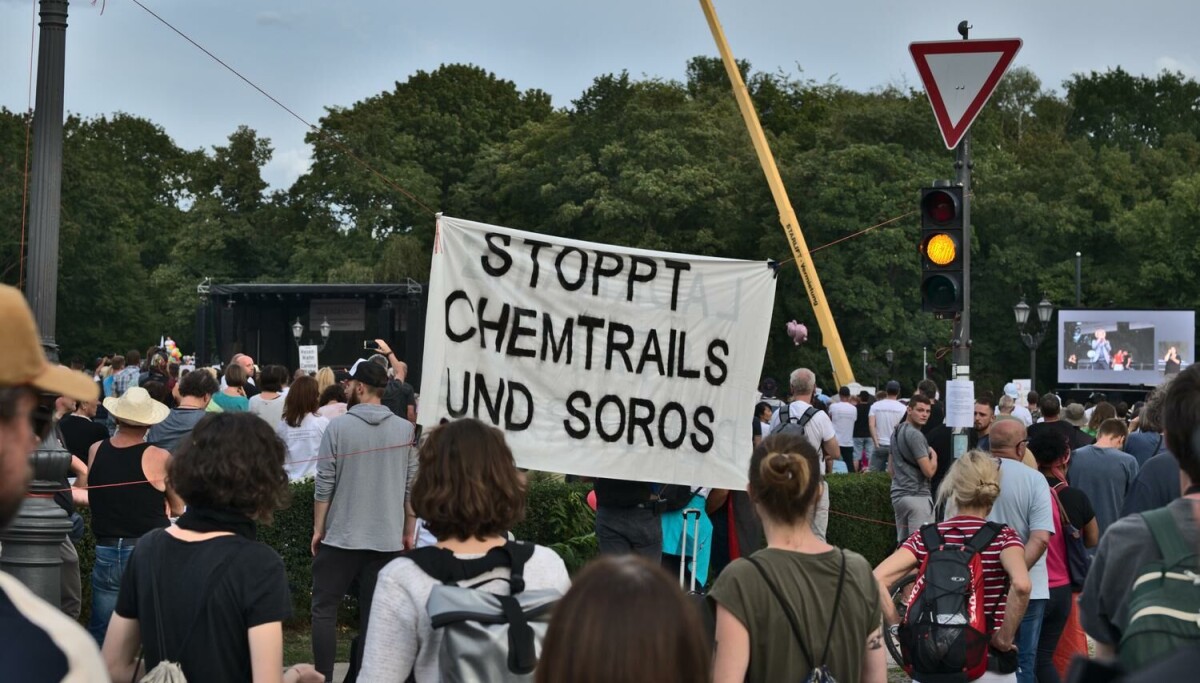This real-life image captures a lively protest scene. The photograph primarily shows the backs of a diverse crowd, all facing toward the center where the protest activity seems to be focused. They are gathered under a makeshift banner strung between a streetlamp and a traffic light, the latter emitting a yellow light. The banner, made of wrinkled cloth, bears the stenciled text "Stop PT chemtrails and Soros." The crowd is a mix of men and women, some with their hair up, some with short hair, and others wearing baseball caps or sunglasses. Attire varies from white shirts and black shirts to striped shirts, with many people carrying backpacks.

In the background, a wall of trees looms, creating a natural backdrop, and above that, a sliver of cloudy or possibly evening sky peeks through. The subtle overcast lighting suggests it is either late in the day or a particularly cloudy afternoon. Notably, behind the crowd to the left, there is a dark green building, though its purpose is unclear. Additionally, a traffic sign with an inverted red-bordered triangle hangs above the traffic light. To the right of the sign, a screen, possibly part of a projector setup or a TV screen, is also visible, although its details are indistinct. The gathering appears substantial, with well over a hundred people participating in this protest.